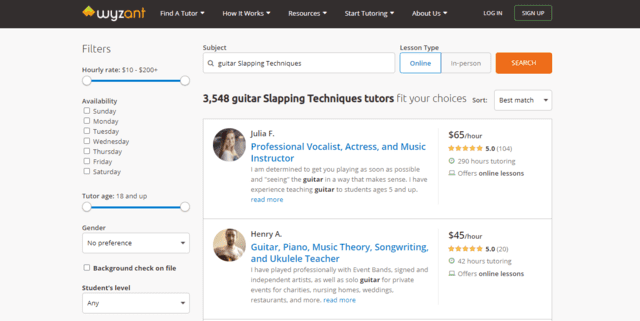The screenshot captures the homepage of the Wysant website, likely accessed from a PC. Wysant is a tutoring platform offering various educational services. 

At the top of the page, multiple navigation tabs are visible, including "Find a Tutor," "How It Works," "Resources," "Start Tutoring," and "About Us." Users can either log in or sign up through the provided links.

Prominently displayed on the site is a search feature accompanied by filters to narrow down the subjects of interest. Currently, the search is set for guitar slapping technique tutors, revealing a substantial pool of 3,548 available instructors.

In the depicted results, two featured tutors are showcased: Julia F. and Henry A. Julia F. specializes in guitar, piano, music theory, songwriting, ukulele, and is also a professional vocalist, actress, and music instructor. Her services are priced at $65 per hour. Henry A. offers tutoring in similar subjects at a rate of $45 per hour. Both tutors boast stellar 5-star ratings, with Julia accumulating 104 reviews and Henry receiving 20.

Additionally, both tutors have accrued significant hours of tutoring experience and provide options for online lessons.